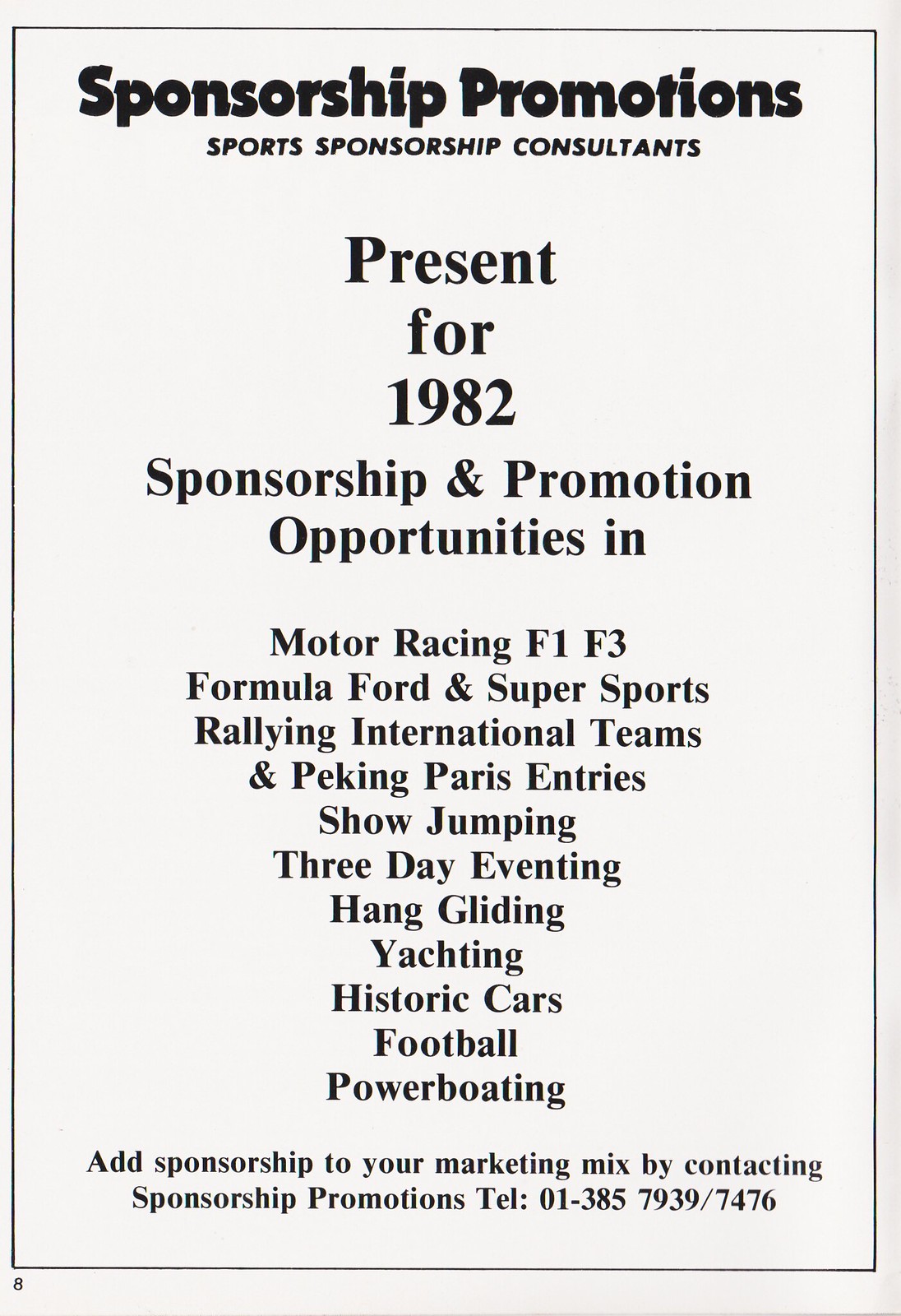This image is a scan of a promotional flyer printed on a white sheet of paper with a thin black border. At the top of the flyer, "Sponsorship Promotions" is prominently displayed in bold black letters. Directly below, in smaller print, it reads "Sports Sponsorship Consultants." The flyer, dated 1982, details sponsorship and promotion opportunities across various sports. It includes categories like Motor Racing (F1, F3, Formula Ford, and Super Sports), Rallying International Teams and Peking Paris Entries, Show Jumping, Three-Day Eventing, Hang Gliding, Yachting, Historic Cars, Football, and Power Boating. Towards the bottom, it encourages adding sponsorship to your marketing mix by contacting Sponsorship Promotions, providing a telephone number: 01-385-7939/7476. Outside the black border, in the lower left-hand corner, the number 8 is visible.